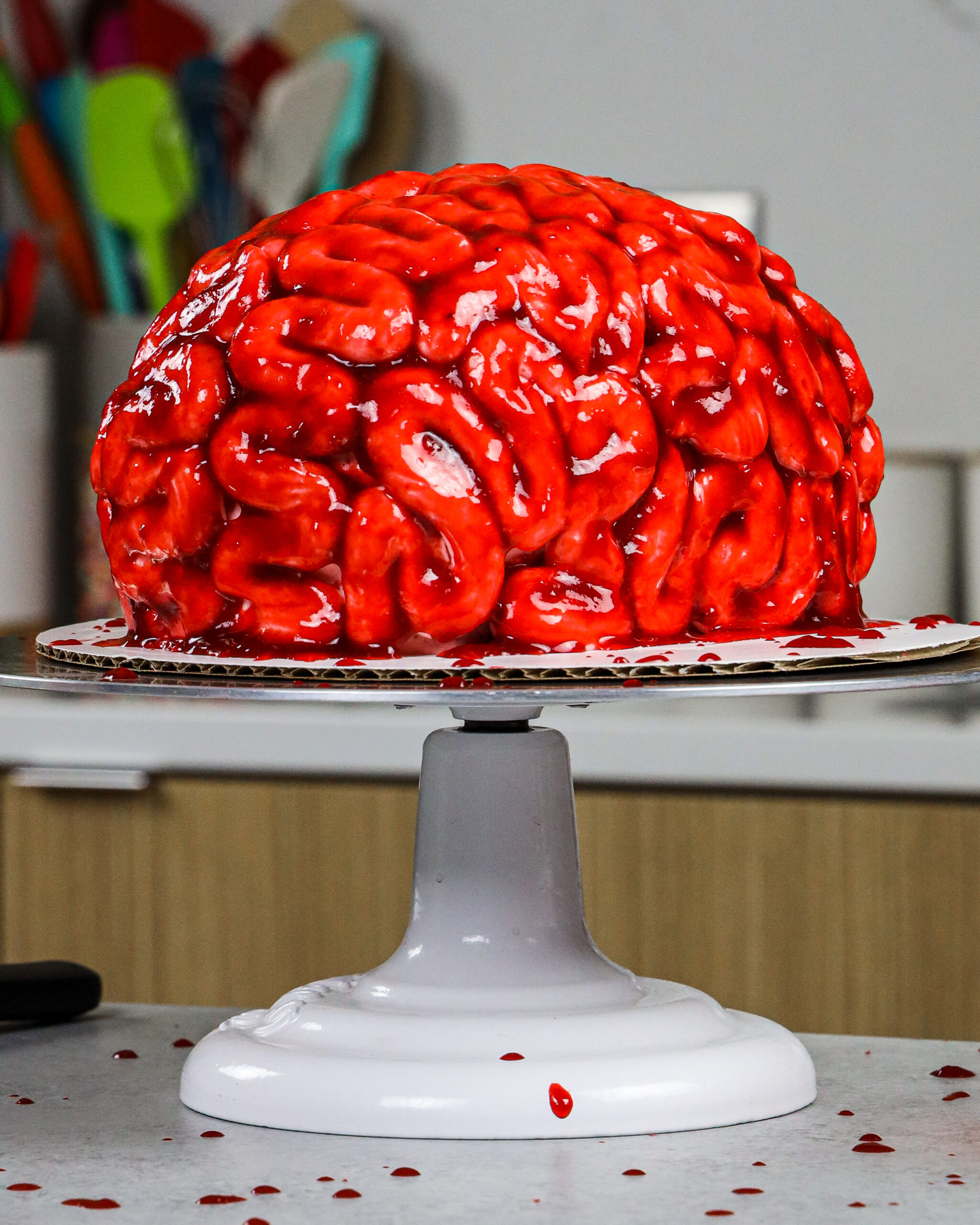The image features a highly realistic cake designed to replicate a human brain, covered in a red, shiny icing that mimics the appearance of blood. This cake sits on a cylindrical cake stand with a wide, circular white base, narrowing before widening again to form a flat plate. Surrounding the base and scattered on the white counter are droplets of red icing, likely from the decoration process. The high-quality portrait photograph captures a detailed view of the cake, complete with intricate zigzags and wiggly patterns, and is set indoors in a kitchen. In the blurred background, there are brightly colored cooking utensils such as whisks and spatulas, adding to the culinary scene. A black, unidentifiable object is also faintly visible amidst the kitchen items, contributing to the authentic atmosphere of the space where this professional or enthusiast cake decorator has crafted their masterpiece.